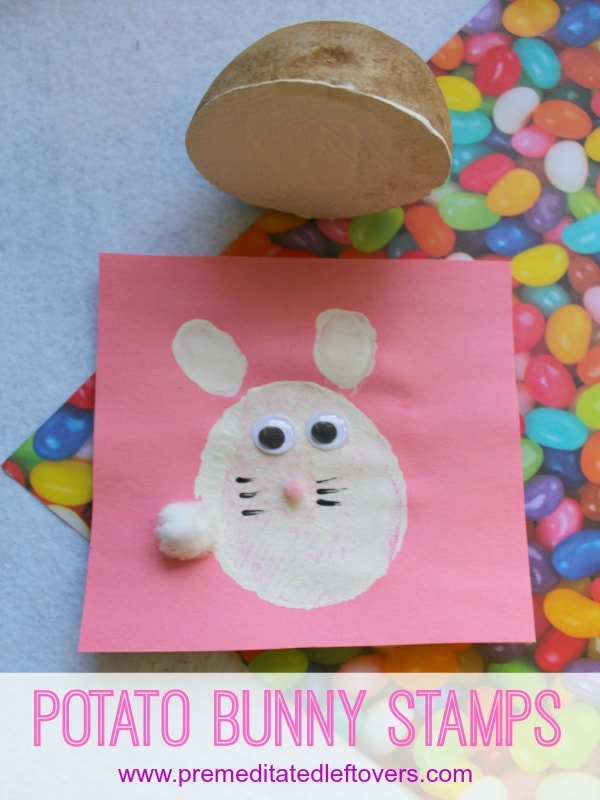The image titled "Potato Bunny Stamps" from www.premeditatedleftovers.com features a detailed and creative Easter-themed artwork. At the top of the image, there is a half potato with brown skin, which appears to have been used as a stamp. This potato has been dipped in white paint. Below the potato, there is a two-layered background; the first layer is a diagonal piece of paper adorned with a vibrant array of colorful jelly beans, displaying colors like pink, orange, white, red, yellow, purple, blue, green, lime green, white, brown, and black. On top of the jelly bean paper, there's a small square pink paper. Central to this pink paper is a stamped figure crafted from the potato, which depicts a bunny. The bunny features a white round body with black eyes, a pink nose, black whiskers, and two white ears formed from fingerprints. Additionally, a piece of cotton serves as the bunny's fluffy tail and another piece for its hand. At the bottom of the image, the text "Potato Bunny Stamps" and the website www.premeditatedleftovers.com are clearly written. The overall composition suggests this image may be part of an advertisement or craft guide for making Easter-inspired potato stamps.